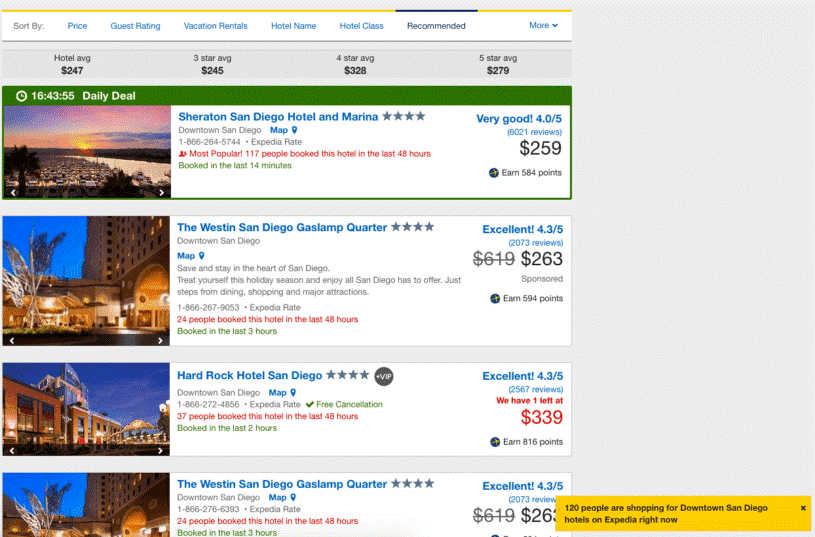Screenshot of a Hotel Booking Page on Expedia: Detailed Overview of Hotel Options in San Diego

This screenshot captures a comprehensive hotel booking page on Expedia, showcasing various hotel options in San Diego complete with their details and pricing. The page features multiple sorting and filtering options such as price, guest rating, vacation rentals, hotel name, hotel class, and recommended.

At the top, an average pricing row displays:
- Overall hotel average price: $247
- Three-star hotels: $245
- Four-star hotels: $328
- Five-star hotels: $279

**Daily Deal Section:**
- **Sheraton San Diego Hotel and Marina:**
  - Classification: 4 stars
  - Location: Downtown San Diego
  - Price: $259
  - Rating: Very good (4.0 out of 5 based on 6,021 reviews)
  - Popularity: 117 bookings in the last 48 hours
  - Recent booking: Last 14 minutes
  - Rewards: Earns 584 points

**Hotel Listings:**
1. **The West End San Diego Gaslamp Quarter:**
   - Classification: 4 stars
   - Location: Downtown San Diego
   - Price: $263 (discounted from $619)
   - Rating: Excellent (4.3 out of 5 stars based on 2,073 reviews)
   - Popularity: 24 bookings in the last 48 hours
   - Recent booking: Last 3 hours
   - Rewards: Earns 584 points

2. **Hard Rock Hotel San Diego:**
   - Classification: 4.5 stars
   - Location: Downtown San Diego
   - Price: $339
   - Rating: Excellent (4.5 out of 5 stars based on 2,567 reviews)
   - Popularity: 37 bookings in the last 48 hours
   - Recent booking: Last 2 hours
   - Rewards: Earns 816 points
   - Additional features: Free cancellation and VIP access

3. (Repeated entry) **The West End San Diego Gaslamp Quarter:** (Details as listed above)

On the right side of the page, a dynamic element indicates that 120 people are currently shopping for downtown San Diego hotels on Expedia. 

Design-wise, the interface is clean with a white background, accented by various colored texts and highlights for emphasis, ensuring ease of navigation and readability.